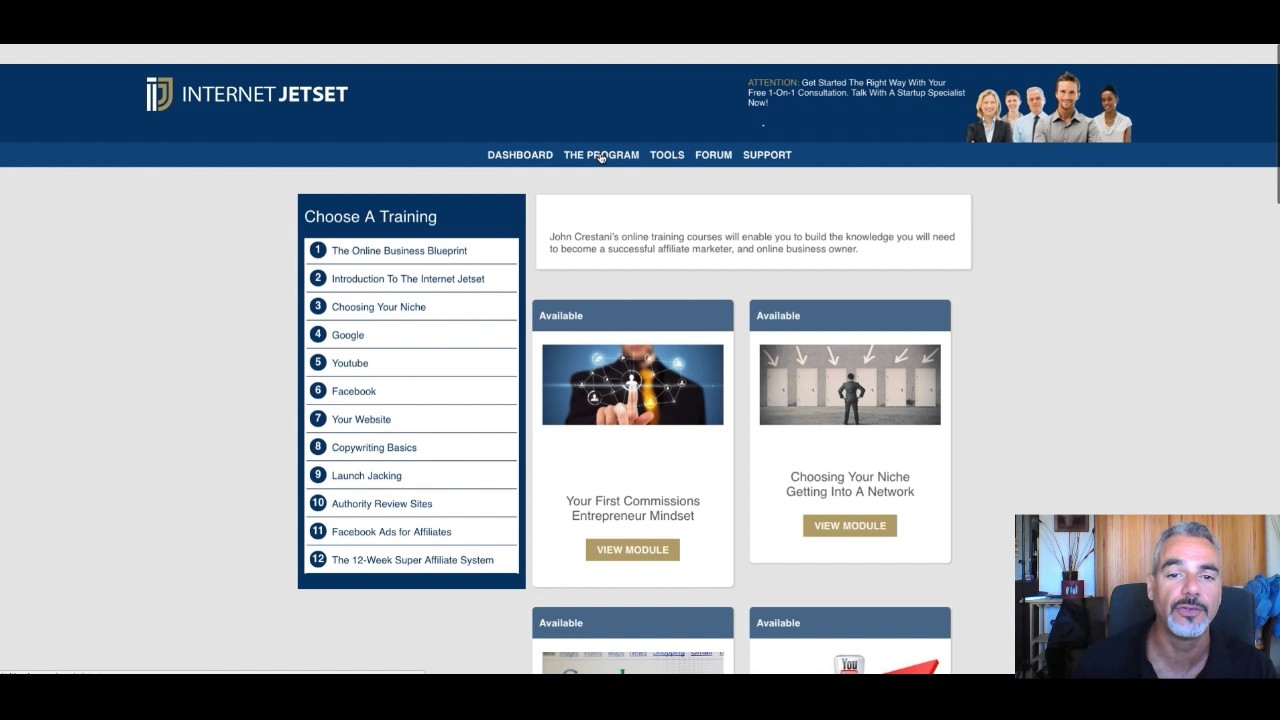A screenshot of a website titled "Internet Jetset," showcasing a dated and seemingly amateur design. The website's header features a stock photo of five people in a typical office setting: two women (one younger and one older), an older man, a younger man, and an African-American woman on the right. The people appear to be Caucasian except for the woman on the right. 

The header includes text that begins with "Attention" and encourages users to "get started the right way," although some details are too small to read clearly. Below the header is a horizontal menu bar with options: Dashboard, The Program, Tools, Forum, and Support. There is also a vertical menu on the left side of the screen listing training modules such as:

- Online Business Blueprint
- Introduction to Internet Jetset
- Choosing Your Niche
- Google
- YouTube
- Facebook
- Your Website
- Copywriting Basics
- Launch Jacking
- Authority Review Sites
- Facebook Ads for Affiliates
- The 12-Week Super Affiliate Program

Several chicklet panels are present, all labeled "available," accompanied by distractingly generic stock photos. One image depicts a man standing in front of six doors with his hands on his hips, another shows a man interacting with 3D computer graphics, and the bottom right corner features a man possibly facing a webcam. The screenshot is bordered by a black bar at the bottom. 

Overall, the layout and design give the website an outdated and cluttered appearance, suggesting a lack of professional polish.